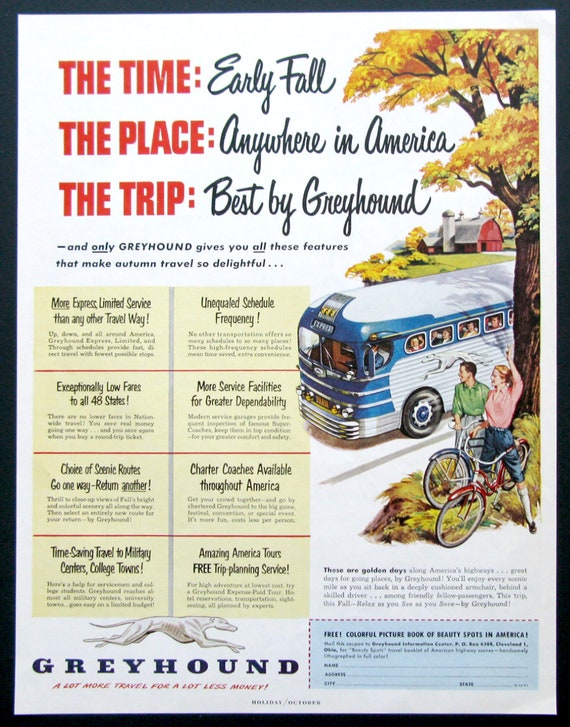The image is an old-timey Greyhound bus advertisement, prominently framed in black with a clean white background. At the top center in bold red text, it reads: "The Time: Early Fall, The Place: Anywhere in America, The Trip: Best by Greyhound." The ad features a nostalgic scene reminiscent of America's yesteryears, possibly set in the 1960s or 1970s. Central to the image is a classic Greyhound bus, adorned with blue paint on the front and a white roof, gleaming under the fall sunlight. Tiny square windows allow a peek at the passengers inside, while a figure in blue, presumably the driver, navigates the bus. Alongside this, a couple, dressed in old-fashioned attire, are depicted on bicycles, cheerfully waving at the passing bus from under a tree with brown trunk and golden autumn leaves.

In the background, a red farmhouse and a suburban cityscape ground the scene in a quintessential American setting. Notably, the right side of the poster includes a graph divided into eight boxes, highlighting various features unique to Greyhound travel. At the bottom, the iconic Greyhound dog logo is placed next to the slogan: "Greyhound: A Lot More Travel for a Lot Less Money." Additionally, the bottom right corner features a coupon offering a free, colorful picture book of beauty spots in America, inviting viewers to enter their name and address to receive it by mail. Above this coupon is a paragraph of small print, adding further details to the advertisement’s offer.